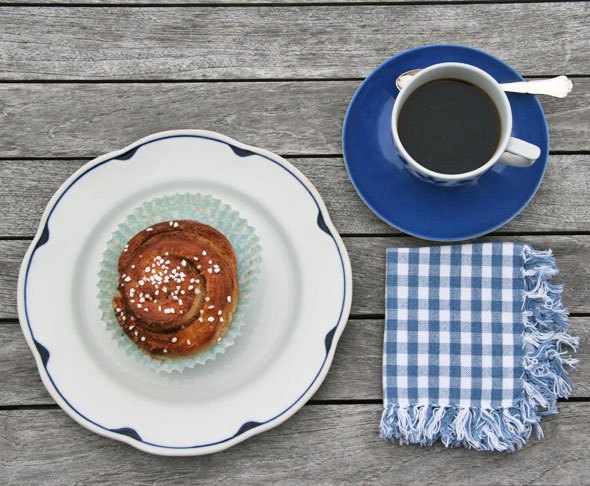The image captures a top-down view of a quaint breakfast scene set on a weathered, grey-slotted wooden table. Central to the composition is a white ceramic plate with a dark blue wavy rim, holding a muffin nestled in a green and yellow cupcake wrapper. The muffin, sprinkled generously with sugar crystals, has a dark brown exterior that spirals inward, resembling a cinnamon roll. To the right, a blue and white checkered cloth napkin is neatly folded, with its fringed edges visible. Above this is a matching blue saucer supporting a white and blue coffee cup, accompanied by a silver spoon resting beside it. The entire arrangement is framed in a landscape orientation, providing a cozy and inviting feel.